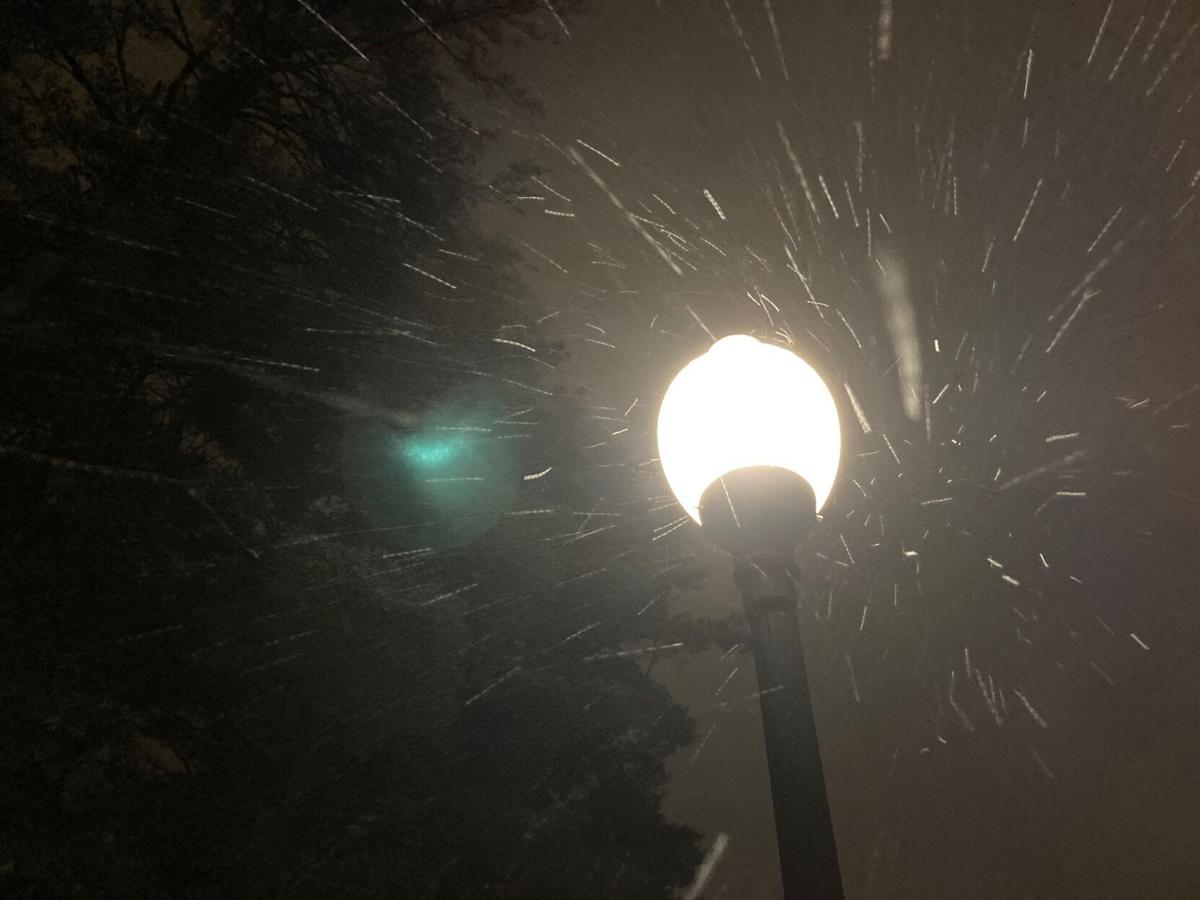This is a nighttime photograph taken from ground level, looking up at an ornate, old-style street lamp with a spherical head that emits a bright, white light. The black pole of the streetlight is lit, and water raindrops, illuminated by the light, appear as white streaks reminiscent of falling pasta. These light streaks extend in multiple directions—vertical, horizontal, and diagonal—adding a dynamic visual effect. To the left of the streetlight, there is a dark green pine tree, partially silhouetted against the black night sky. Additionally, a teal lens flare is visible to the left of the lamp, with the sky appearing dark gray due to the lighting. The scene is captured during a rain shower, emphasizing the ambiance of a rainy, nighttime cityscape.